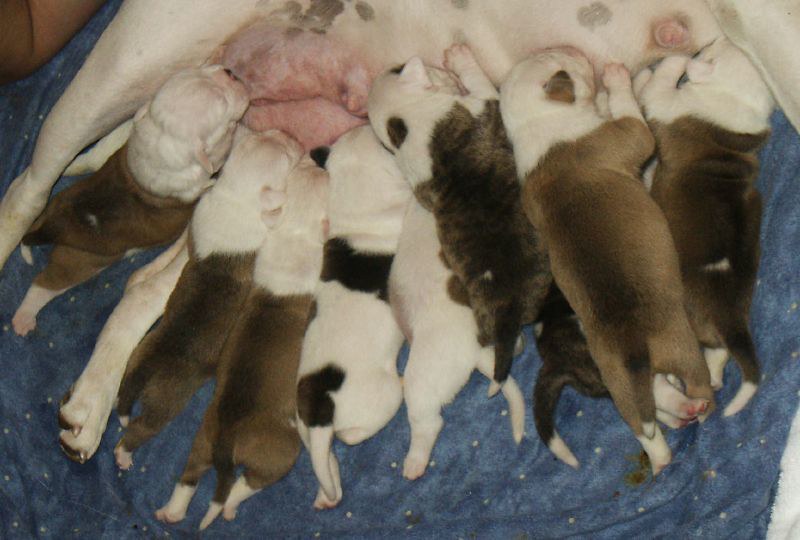In this color photograph, a mother British Bulldog is feeding her eight newborn puppies on a blue blanket. The close-up image focuses on the mother's belly and teats, with only traces of one of her forelegs visible. The eight puppies have varying fur patterns; three on the left have white heads with grey and brown bodies, two in the middle are white with distinct brown spots on their backs and legs, and the remaining three on the right have white heads with brown and grey bodies. One of these rightmost puppies is notable for a spot on its head. All the puppies, appearing no more than a few days old, are energetically nursing from their mother. The simplistic backdrop emphasizes the tender moment without any additional distractions such as writing, people, plants, or structures.